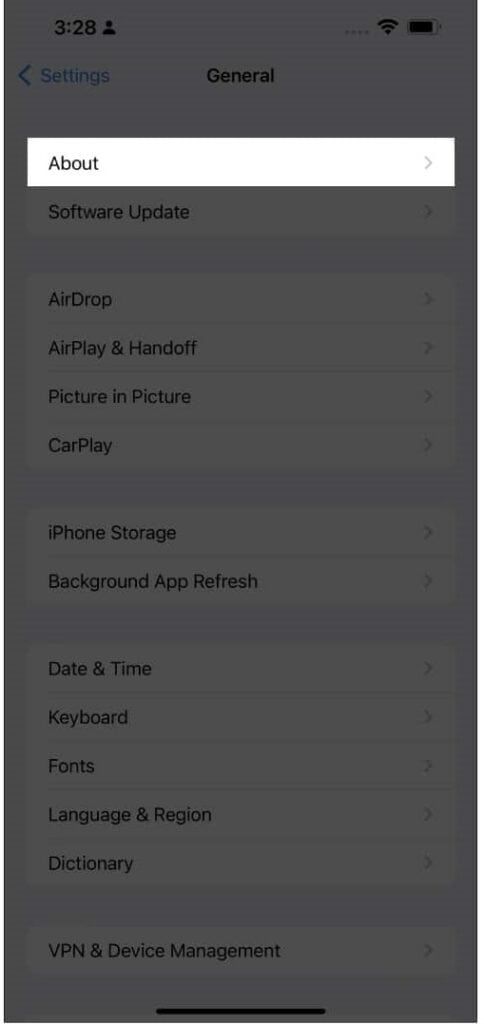The image displays a smartphone screenshot with the time shown as 3:28 at the top left, next to black Wi-Fi and badge icons on the top right. The phone's background is white. 

On the screen, a menu labeled "About" is selected and prominently displayed in black text on a white background at the top, appearing to pop up. The rest of the settings menu is visible but tinted.

Just above the "About" section, the heading "General" is indicated in black text, accessed through the "Settings" menu, which is marked in blue text with a back arrow icon pointing left, also blue, at the top left of the screen. 

Below "About," the following menu options are listed:
- Software Update
- AirDrop
- AirPlay & Handoff
- Picture in Picture
- CarPlay
- iPhone Storage
- Background App Refresh
- Date & Time
- Keyboard
- Fonts
- Language & Region
- Dictionary
- VPN & Device Management